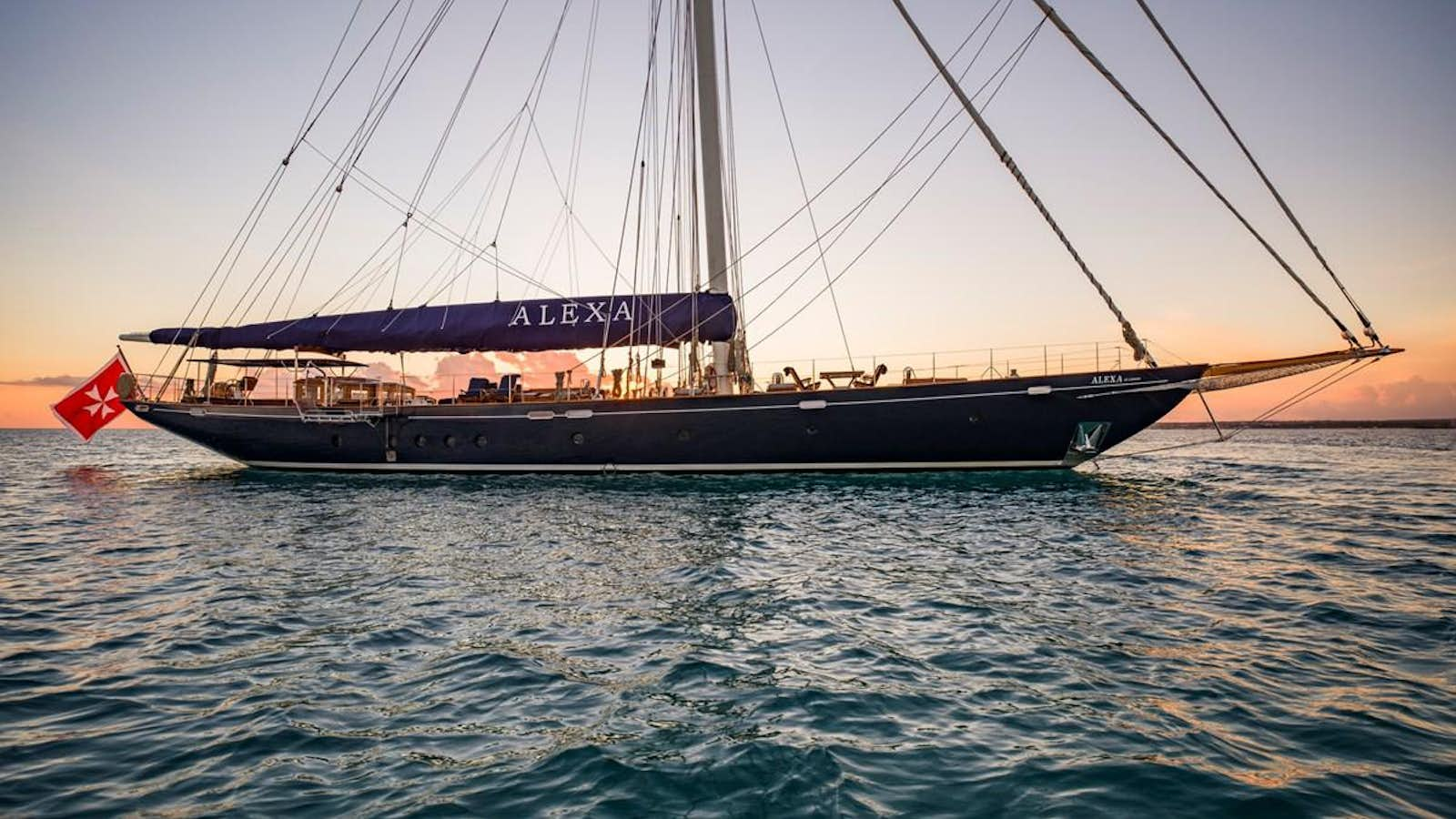The photo captures a tranquil scene at sunset on the water, with a large, elongated sailboat centered in the image. The dark blue, nearly black hull of the boat is accented by a white pinstripe and dotted with small, round windows. The sleek vessel, identified as "Alexa" by the white lettering on its side, has its sails rolled up and covered with a blue material, rendering the mast and numerous supporting ropes strikingly visible. At the rear of the boat, a distinctive red flag with a white cross composed of inward-pointing arrows is prominently displayed. The surroundings show a calm body of water, likely an ocean, with the sun having just set, coloring the horizon in shades of orange and yellow that gradually transition to a bluish-gray sky. The few scattered clouds at the horizon's edge are tinged with a faint red hue, further enhancing the serene, picturesque atmosphere of the scene.